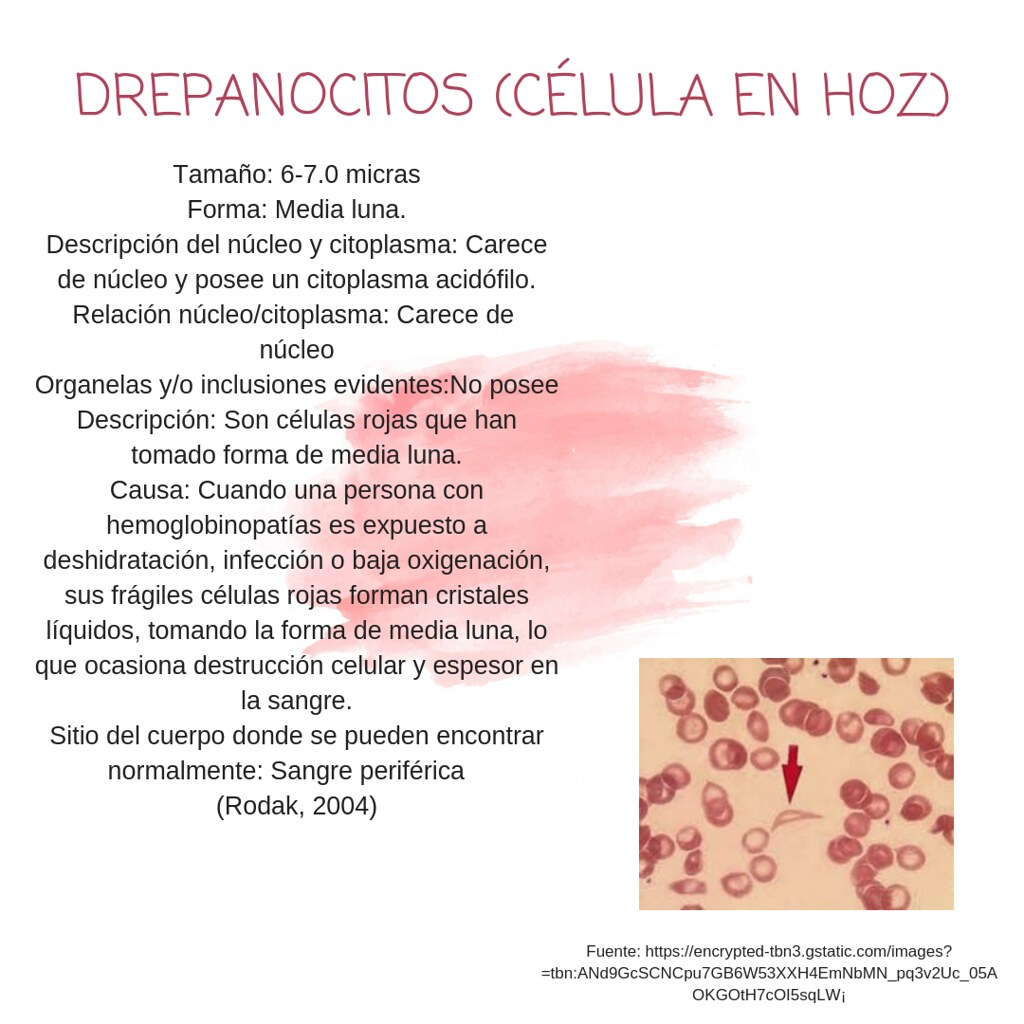The image depicts a detailed medical document written in a foreign language, likely Portuguese. It features black typed lines on a white background and prominently displays a reddish-pink smudge in the center, possibly a paint or blood stain. At the top, in dark pink text, the title reads "Drepanoctyos, Cellula, Hose". Towards the bottom right, there is a microscopic photograph showcasing pink cells against a peach or cream background, with a red arrow pointing to a misshapen cell, resembling a sickle cell. Surrounding the misshapen cell are numerous small red circles, likely representing other cells. Additionally, the text references "Rodak, 2004" at the very end, providing context for the medical content displayed in the document.